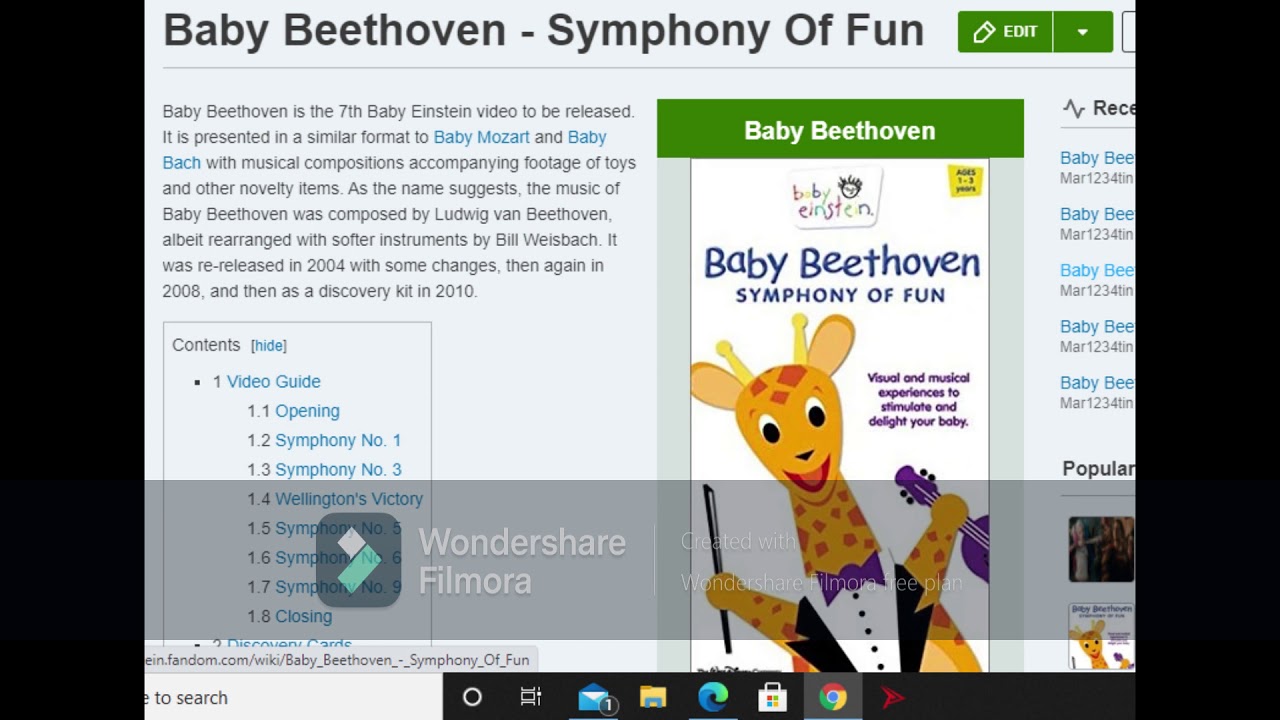A screenshot from what appears to be a wiki page, specifically an article about "Baby Beethoven: Symphony of Fun." The page features a navigation area showcasing an article summary and selectable contents for easy navigation. On the right side of the screen, there's an image depicting a joyful, cartoon-like giraffe holding a violin and bow, looking directly at the viewer. The image caption describes visual and musical experiences designed to stimulate and delight young audiences.

The introductory section notes that "Baby Beethoven" is the seventh video in the Baby Einstein series, following the same format as previous releases. The music, composed by Beethoven, is arranged with softer instruments by Bill Weisbach. The video was initially released in an unspecified year, then re-released with modifications in 2004, again in 2008, and as a Discovery Kit in 2010. The article features a light gray background, differing from Wikipedia's standard white backdrop.